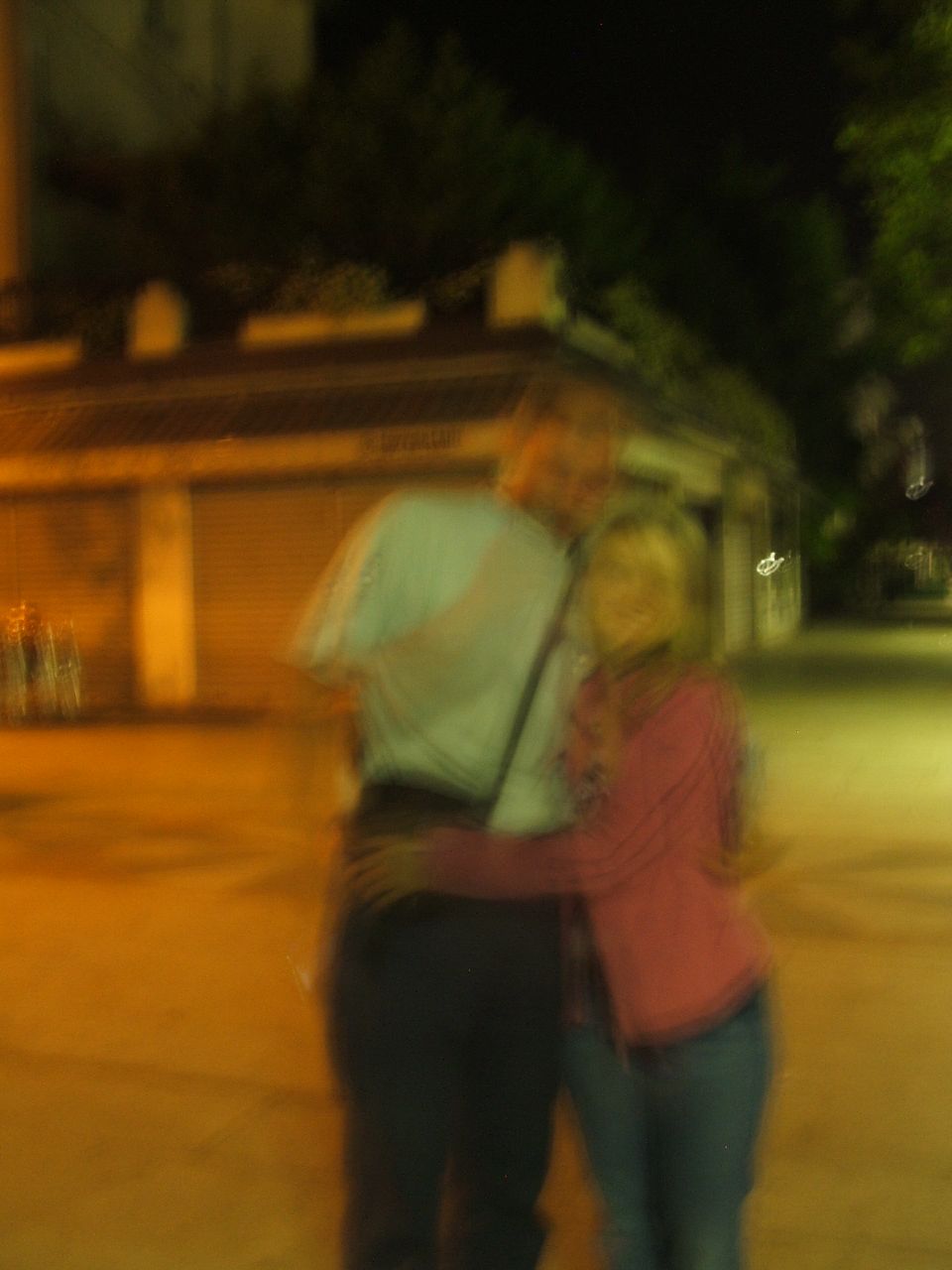This is a very blurry nighttime photograph depicting a man and a woman standing in an embrace on a street illuminated by incandescent orange streetlights. The man, who is wearing a white t-shirt and dark pants, stands with his arm around the woman's waist, while the woman, dressed in a pink sweater and blue jeans, wraps her arms around his waist in return. The woman has dirty blonde hair. They appear to be smiling at the camera, although their faces are indiscernible due to the blur. Behind them is a building with a closed garage and a long stretch of pavement leading toward it, and beyond the garage, trees and foliage can be seen.